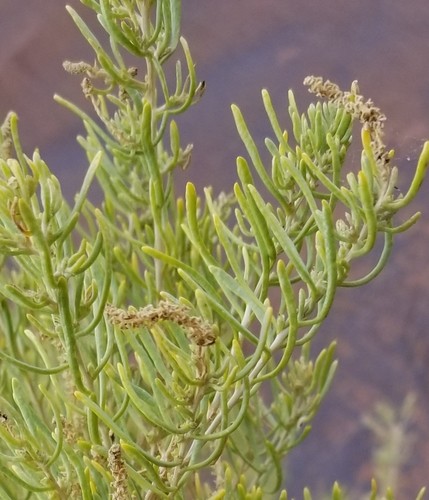The photograph captures a close-up of a unique, noodle-like stemmed plant that dominates the frame, radiating a vibrant green hue with yellowish-green tips. The central stems curve elegantly, branching off into numerous thin, needle-like leaves that extend outwards in various directions—vertically, horizontally, and diagonally. Some of these stems culminate in light brown, bulbous or seeding formations, indicating a state of partial desiccation. The background, a blurred haze of light purple interspersed with shades of brown and gray, creates a contrasting backdrop that emphasizes the plant's structure. This haziness hints at mountainous or dry vegetation but remains indistinct, ensuring the plant remains the focal point of the image. The overall composition evokes the resilience of vegetation in arid climates, reminiscent of the persistent, repetitive forms found in such environments.